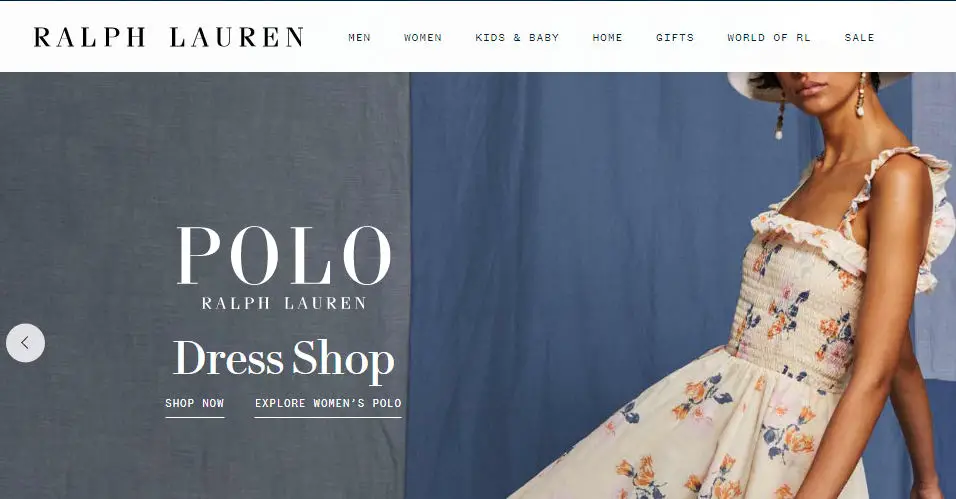This screenshot showcases the homepage of the Ralph Lauren website. At the top of the image, a black header displays the "Ralph Lauren" logo on the left side, followed by navigational categories: Men, Women, Kids & Baby, Home, Gifts, World of RL, and Sale. Beneath the header, the left section of the page features a large promotional image with a gray background. Text overlaying this background reads "Polo Ralph Lauren Dress Shop," along with two interactive hyperlinks: "Shop Now" and "Explore Women's Polo," all in white font.

On the right side of the image, the background changes to a rich blue, resembling draped fabric. A woman is partially visible, wearing a white hat and earrings. Her face is mostly cut off, leaving just a portion visible. She is dressed in a cream-colored, tea-length dress adorned with ruched detailing in the front, a ruffled neckline, and ruffle straps at the shoulders. The dress flares out from the bodice and features a spaced-out floral print in shades of blue, yellow, red, and pink. The woman is posed with her body angled to the left while her face looks directly ahead, showcasing her elegant attire in a detailed and visually appealing manner.